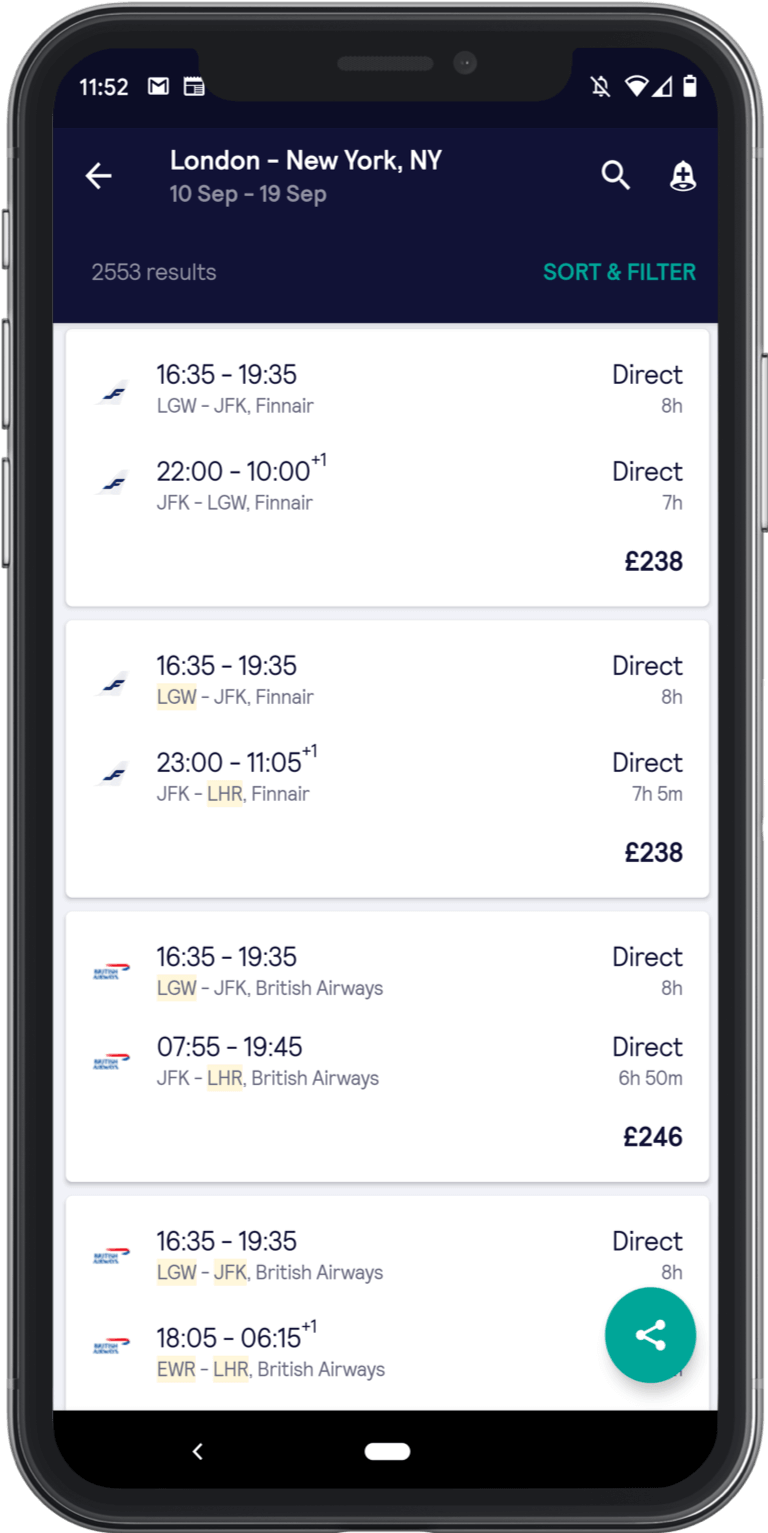The image depicts a smartphone screen displaying a flight search interface. The device shows the current time as 11:52 AM, located at the top left corner. Several status icons are visible: an email icon indicating a notification, a calendar symbol, muted sound, a half-full Wi-Fi signal, a mobile network signal at half strength, and a battery icon showing approximately 75% charge.

The search details are focused on flights from London to New York, set for departure on September 10th and return on September 19th, yielding 2,553 search results. The first listed flight departs at 10:35 and arrives at 19:35, with a noted duration of three hours. Despite the varying departure and arrival times due to time zone changes, the flight is marked as being between 10 PM and 10 AM, both as direct flights. The first flight costs 238 Euros, and is operated by Finnair. Another option from the same airline departs at 11 PM and arrives at 11:05 AM, also priced at 238 Euros.

Other options include flights with British Airways. The first option departs at 16:35, arriving at 19:35, with the second leg leaving at 07:55 AM and arriving at 19:45 PM, costing 246 Euros. A subsequent British Airways flight departs at the same early time but lands at 06:06 PM, with no visible price—presumably similar to the others.